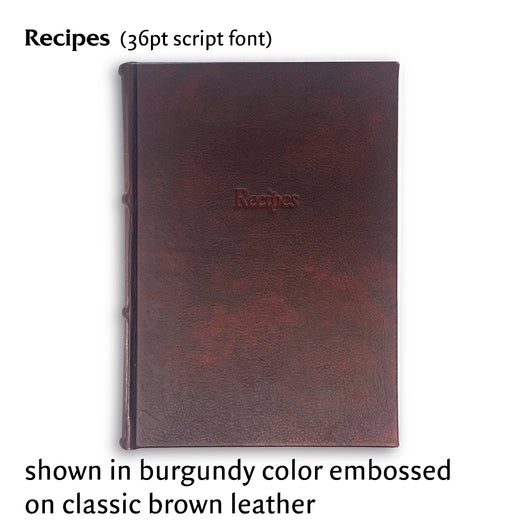The image is a color photograph of a promotional picture showcasing a leather-bound book intended for sale. Centered on a white background, the closed book appears to be made of dark, rusty brown leather. Embossed in the middle of the cover is the word "Recipes." Surrounding the book, additional black text provides details: at the top, it reads "Recipes" in a 36-point script font, and at the bottom, "Shown in burgundy color, embossed on classic brown leather." The overall presentation of the image is designed to give prospective buyers a clear view of the product's quality and appearance, highlighting its elegant and classic style.